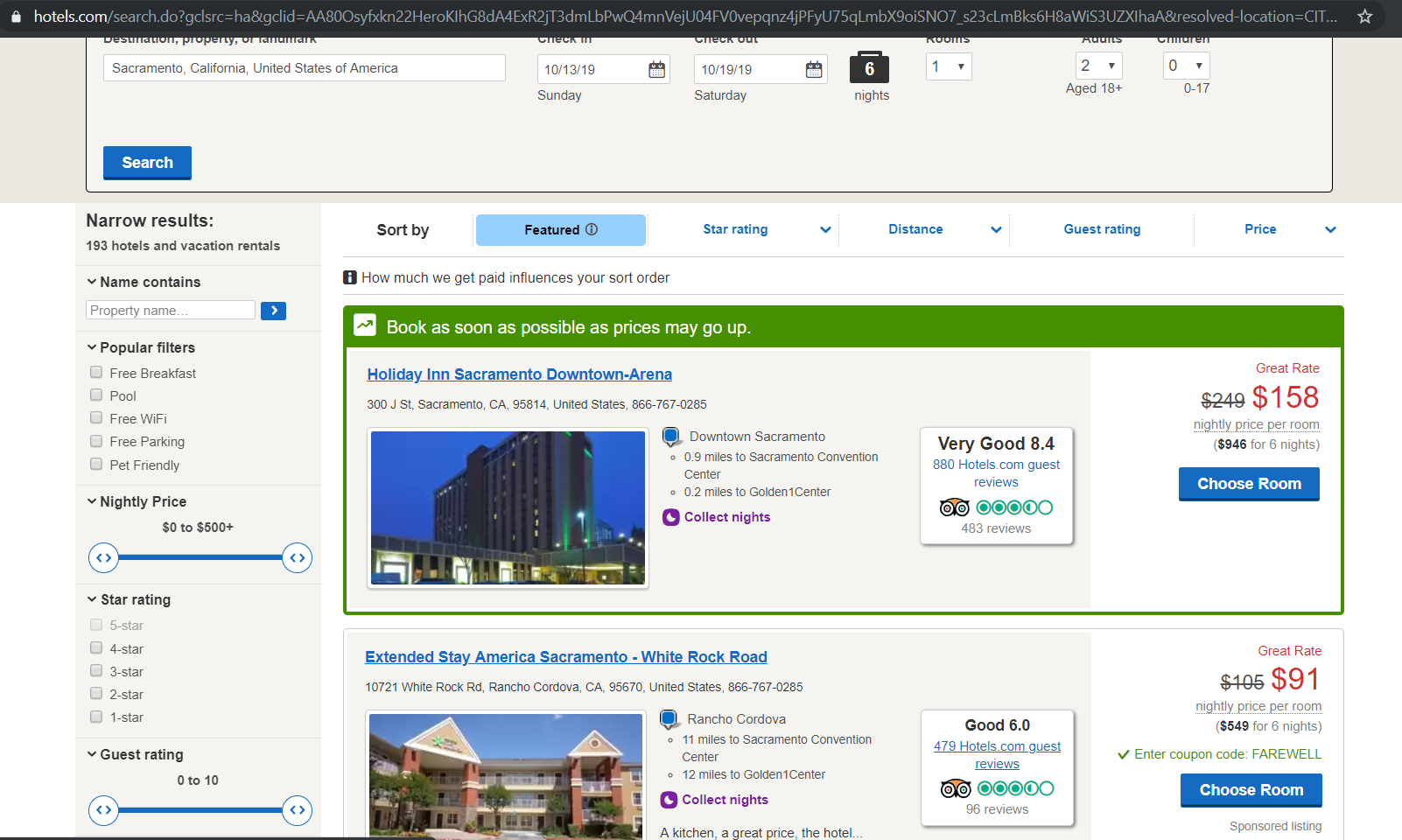**Screenshot Description: Detailed Hotel Booking Website Search**

The screenshot captures a webpage from Hotels.com, illustrating the results of a hotel search. The address bar at the top shows the URL of the site. The search criteria specified includes the destination, Sacramento, California, United States, with check-in on Sunday, October 13, 2019, and check-out on Saturday, October 19, 2019, for a total of six nights. The booking is for one room accommodating two adults (18+), with no children. A blue "Search" button is displayed below these details.

On the left-hand side of the screen, additional search filters can be applied. The filters include:
- **Property Name Search**: Allows input of a specific property name with a blue search arrow.
- **Popular Filters**: Options for free breakfast, pool, free WiFi, free parking, and pet-friendly properties, none of which are selected.
- **Nightly Price Range**: Adjustable bar from $0 to $500+.
- **Star Rating**: Options ranging from one to five stars, none of which are selected.
- **Guest Rating**: Adjustable bar for guest ratings from 0 to 10.

In the middle section, sort options are available, which include:
- **Sort By**: Featured, with further selections for star rating, distance, guest rating, and price.
Additional notices: "How much we get paid influences your sort order" and "Book as soon as possible as prices may go up."

**Hotel Listings**:

1. **Holiday Inn Sacramento Downtown-Arena**
   - **Address**: 300 J Street, Sacramento, California, 95814, United States
   - **Contact**: 856-767-0285
   - **Proximity**:
     - 0.9 miles to Sacramento Convention Center
     - 0.2 miles to Golden One Center
   - **Reviews**:
     - Very Good - 8.4/10 from 880 Hotels.com guest reviews
     - 483 reviews from Trustpilot
   - **Price**:
     - Original rate: $249, on sale for $158 per night
     - Total for six nights: $946
   - **Additional Information**: Collect nights, choose room option displayed via a blue button.
   - **Image**: A picture of the hotel is provided adjacent to these details.

2. **Extended Stay America Sacramento - White Rock Road**
   - **Address**: 10721 White Rock Road, Rancho Cordova, California, 95670, United States
   - **Contact**: 866-767-0285
   - **Proximity**:
     - 11 miles to Sacramento Convention Center
     - 12 miles to Golden One Center
   - **Reviews**:
     - Good - 6.0/10 from 479 Hotels.com guest reviews
     - 96 reviews from Trustpilot
   - **Price**:
     - Original rate: $105, on sale for $91 per night
     - Total for six nights: $549
   - **Promotion**: "Enter coupon code FAREWELL"
   - **Additional Information**: Sponsored listing, a snippet of hotel amenities mentions a kitchen and great price, though some text is obscured.
   - **Image**: An accompanying photo of the hotel is partially visible.

Both listings feature blue "Choose Room" buttons for further booking actions.